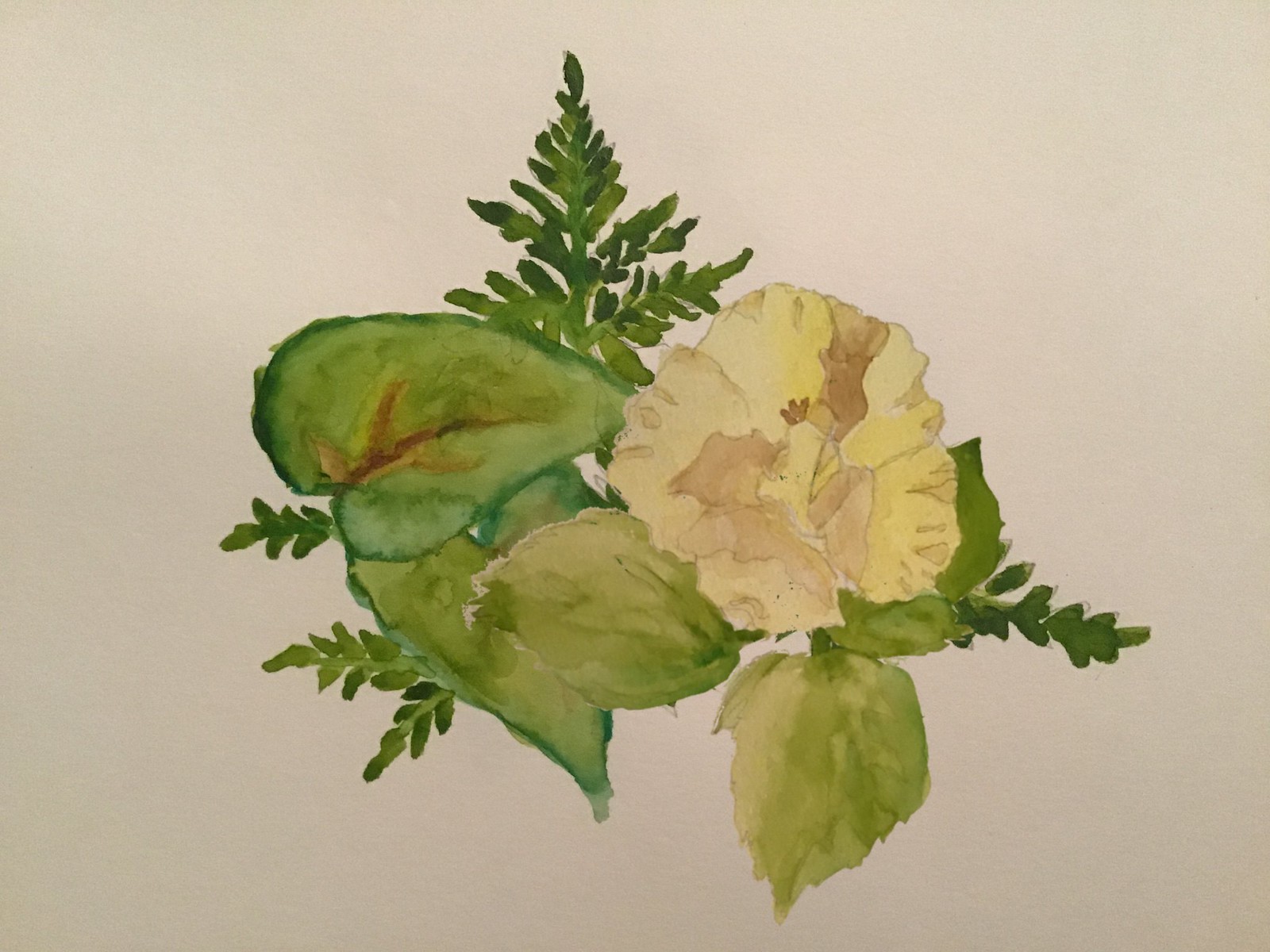This is a delicate watercolor painting on white paper, featuring a vibrant floral and foliage composition. Central to the artwork is a stylized flower resembling an iris, rendered in shades of yellow and brown. Surrounding the flower is a cluster of small, fern-like greenery, adding an intricate layer of detail. Interspersed among the foliage are two distinctive leaves that appear to be from a pothos ivy, their rich forest green hues subtly accented with touches of yellow. The overall color palette enhances the delicate, translucent quality typical of watercolor paintings. This detailed and harmonious illustration exudes an elegant simplicity, capturing the natural beauty of the plants in a gentle, artistic manner.